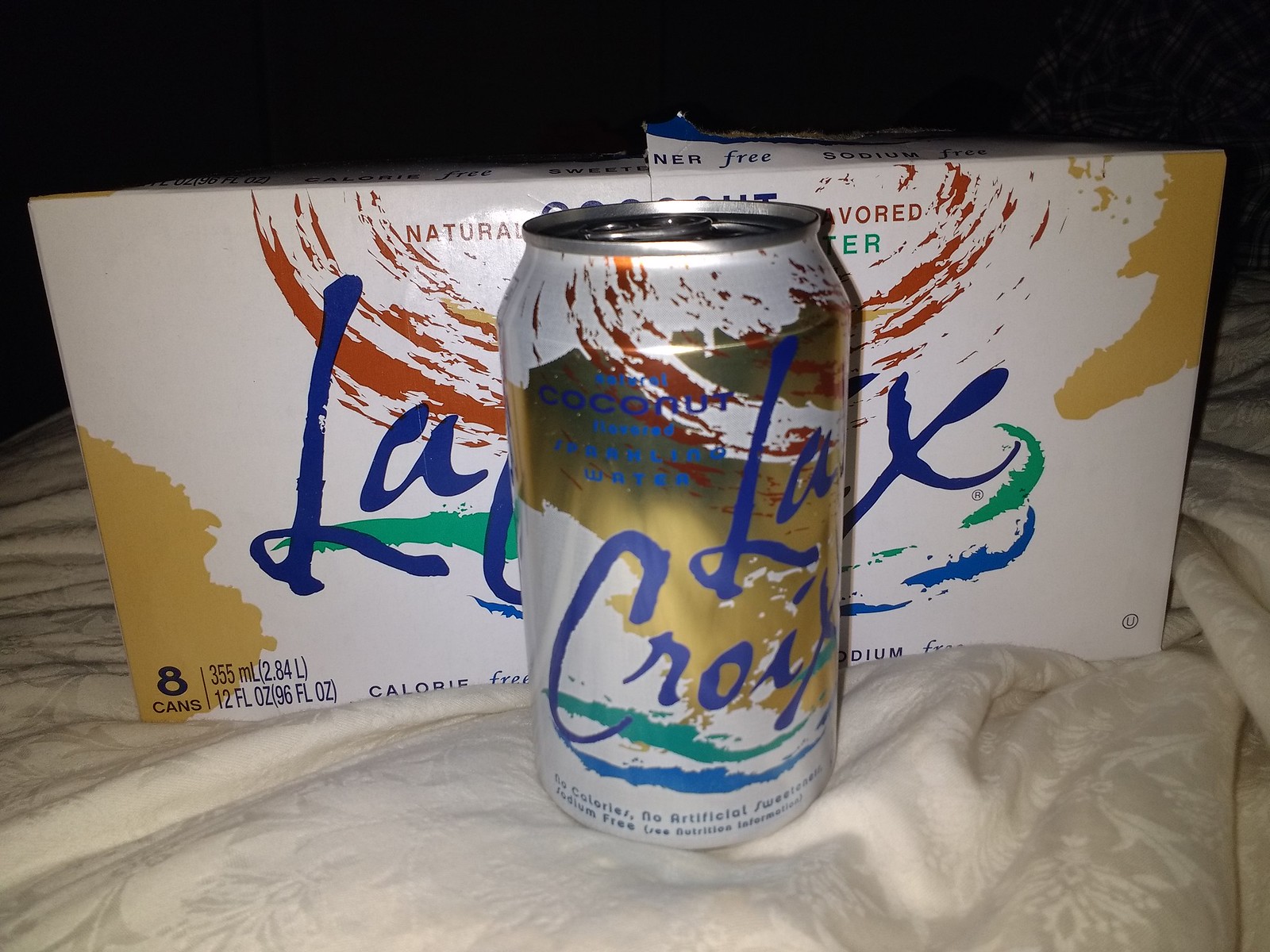A dimly lit room with a black background highlights a scene where a white sheet of fabric is draped, adorned with various plants and flowers. In the foreground, there is a white can featuring a prominent gold medal emblem. The can is embellished with bright blue and red elements, along with green accents at the bottom. Amidst this arrangement, a hand-drawn green box is visible in the background, indicating measurements of the can: 5 milliliters, 2.4 milliliters, 12 fluid ounces, and 9.6 fluid ounces. The text on the can is displayed in a striking blue color.